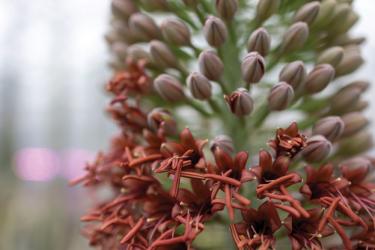This close-up photograph captures a unique and intriguing plant that appears to belong to a desert-dwelling species. The plant features a central green stem from which multiple smaller stems extend. Each smaller stem ends in buds that resemble miniature tulips. The photograph shows a striking contrast between the top and bottom halves of the plant. In the upper portion, the buds are tightly closed, displaying a light pale pink or dusty pink color. These unopened buds contribute to the plant's conical overall shape.

In contrast, the lower section of the plant reveals buds that have burst open, revealing stick-like petals in a rust burnt sienna or amber color. These open blossoms have a tubular shape, distinct from traditional flower petals. The background is blurred out completely, appearing white and hazy, which isolates the plant in sharp focus and emphasizes its details. Additionally, there are indistinguishable pinkish lights visible on the left-hand side of the image. This coloration and the blurred background give the image a somewhat cold and wintry feel, further accentuating the unusual and captivating appearance of the plant.